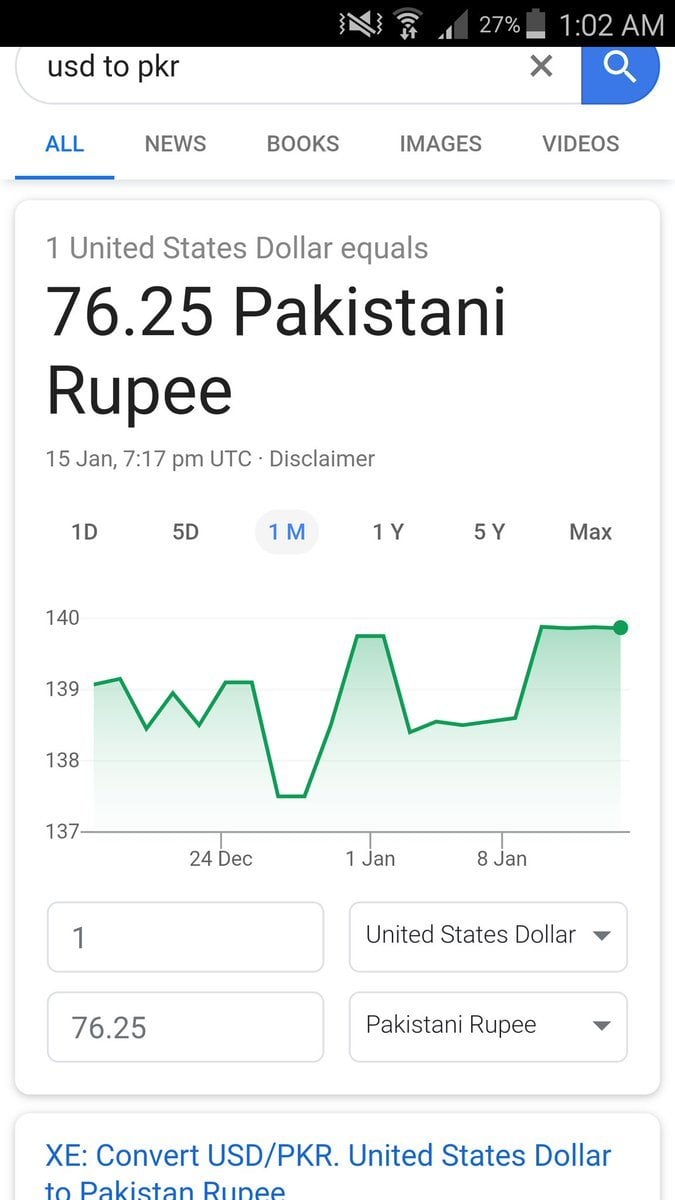The image is a vertical screenshot captured from a smartphone device, with a predominantly white background likely emanating from a computer screen. At the top of the image, there is a black rectangular strip housing various status icons. From left to right, these icons include a muted sound symbol, a Wi-Fi signal accompanied by up and down arrows, a partially filled triangle, an indication of 27% battery life, and the timestamp, 1:02 a.m.

Beneath this strip, there is a white search bar displaying the query "USD to PKR". Located within the bar are a gray 'X' for clearing the search, and a blue box featuring a magnifying glass icon used to initiate the search. The highlighted text in blue indicates that the user has selected the 'All' tab, although there are other tab options available such as News, Books, Images, and Videos.

The subsequent section presents the search results. It begins with the information that "1 United States dollar equals 76.25 Pakistani rupees", displayed in gray and black text respectively. This data is timestamped with "15th of January, 7:17 p.m. UTC" and includes a 'Disclaimer' note. There are also time frame options highlighted in blue, allowing the user to view exchange rates over different periods—one day, five days, one month, one year, five years, and maximum available data.

A green line graph appears next, depicting the fluctuations in the exchange rate over the selected time frame, marked with various dates and corresponding exchange values.

At the bottom of the image, there is a blue hyperlink labeled "XE convert USD to PKR—United States dollar to Pakistani rupee," indicating an option to perform a currency conversion on the XE platform.

This detailed screenshot provides a comprehensive overview of the real-time exchange rate between the United States dollar and the Pakistani rupee, complete with graphical data and additional resources for further information.